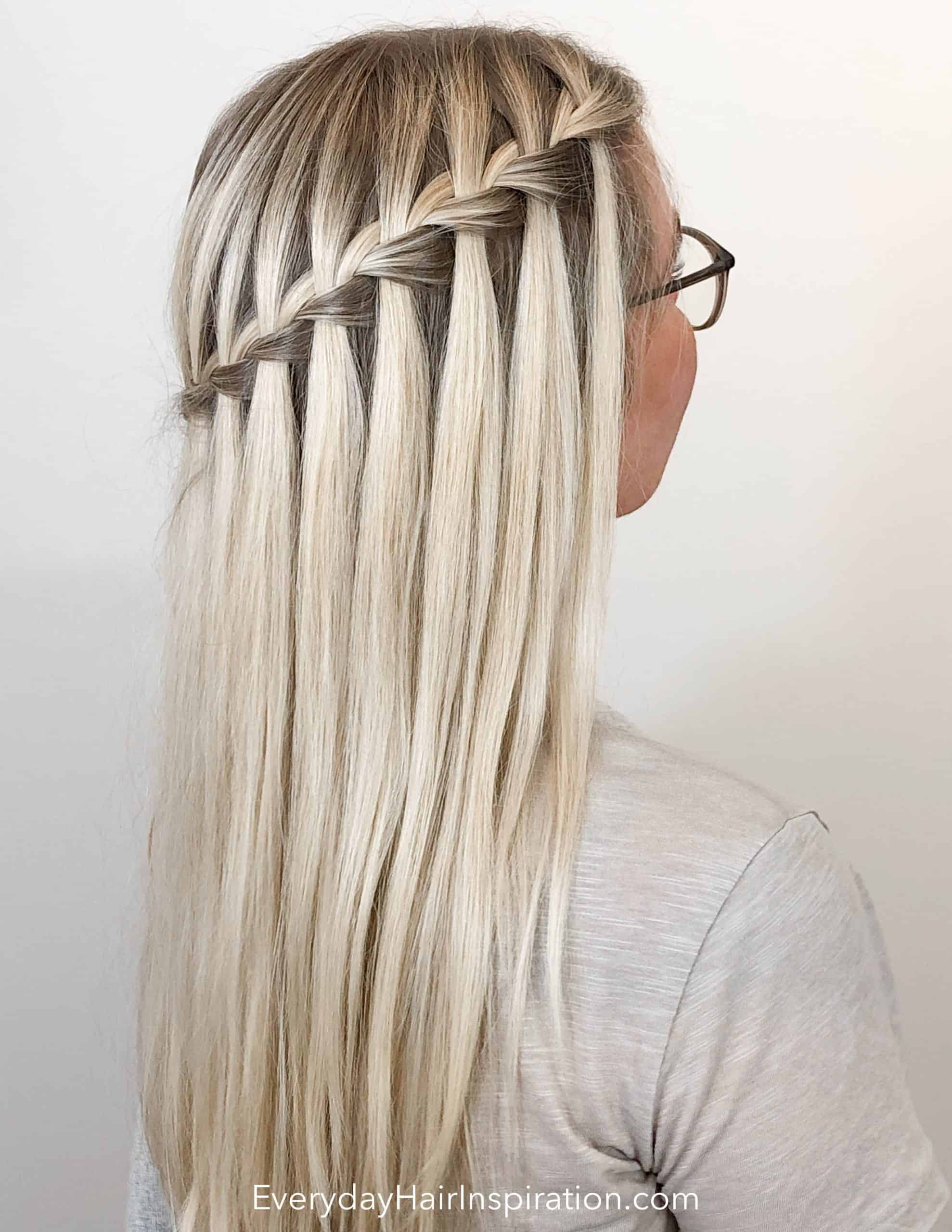This photograph features a Caucasian woman standing in front of a plain white wall, with the focus squarely on her intricate hairdo. Her long blonde hair, accented by dark roots, is styled in a diagonal braid that begins at the top right of her head and elegantly sweeps down to the bottom left. She is wearing dark brown, possibly tortoiseshell, glasses, and a burnout pattern t-shirt that is white or light gray. Notably, she appears to be wearing no makeup. At the bottom of the image, a white watermark reads "everydayhairinspiration.com."